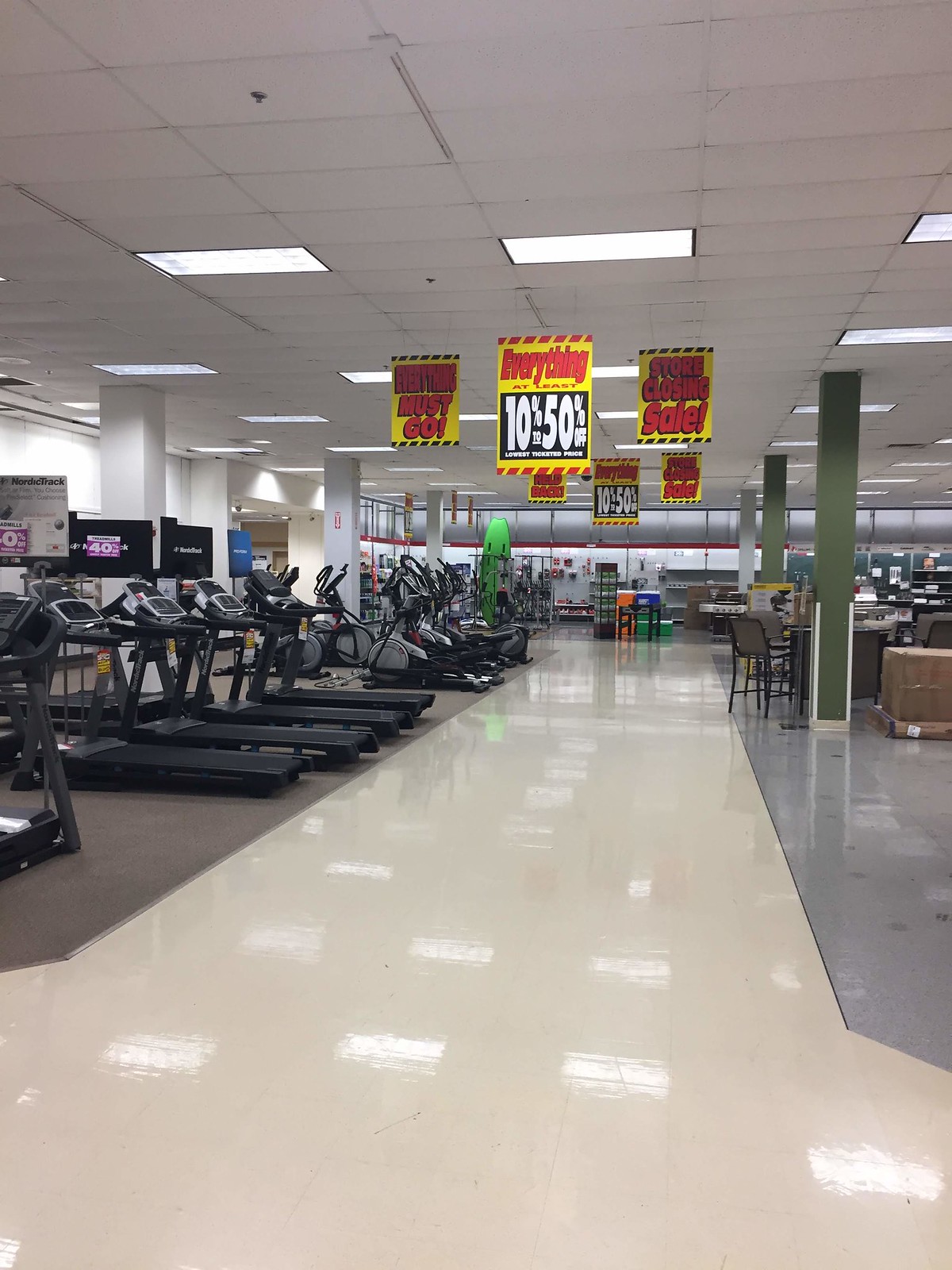The photograph showcases the interior of a retail store, featuring a long, gleaming white linoleum floor that reflects the overhead fluorescent lights embedded in the ceiling tiles. On the right side of the frame, the floor transitions to a gray surface, extending out of view. To the left, a section of flat gray carpet accommodates several black treadmills, neatly aligned. Suspended from the ceiling above the treadmills are eye-catching gold signs with red print, announcing discounts of 10% to 50% off, with the specific percentages highlighted in white on a black background. Additional gold and red signs proclaim a "Store Closing Sale" with the decisive statement "Everything Must Go."